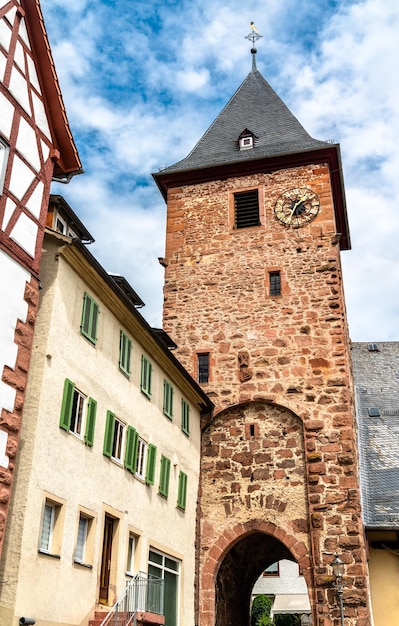The photograph captures a very tall and imposing brick tower centrally located among adjacent buildings. The tower, constructed from red and brown bricks, features an archway with a brick-edged entrance at its base. As the eye moves upward, several small windows punctuate the tower's height. Just below the roof, there is an analog clock positioned on the right side of the structure. The roof is a striking red and pointy, crowned with a weather vane and featuring a small window at its center.

Adjacent to the tower, a three-story beige building with green shutters sits perpendicular to it, serving as a housing unit. Another taller building, attached to this housing unit, is visible on the left. The skies above are a clear blue interspersed with a few clouds, adding to the serene atmosphere of the scene.